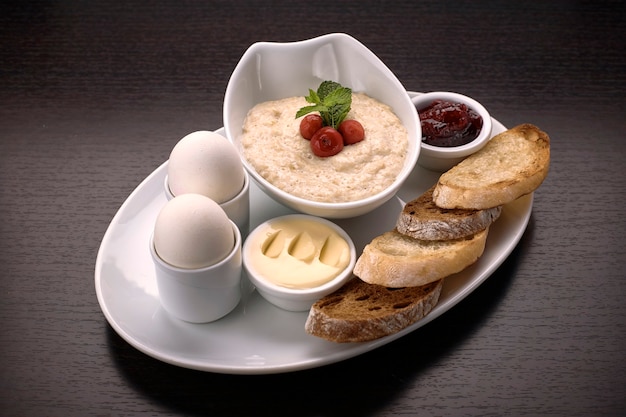The image showcases a meticulously arranged white oval plate filled with an assortment of breakfast foods, centered on a brown, horizontally grooved wooden table. On the left side of the plate, two white egg holders each cradle a hard-boiled egg, their pristine shells uncracked. Beside these stands a pair of small bowls, one containing a beige pudding-like substance and the other holding a bit of pale yellow butter. A larger central bowl contains what appears to be creamy oatmeal or porridge, garnished with bright red tomatoes, adding a touch of freshness and color. To the right, a smaller bowl brims with a deep purple jam or jelly. Completing the ensemble, below these various bowls and still on the plate, rest four pieces of crusty, toasted bread — two made from rye and the other two from white bread — perfectly sized for dipping into the surrounding delicacies. The overall impression is of a thoughtfully prepared, visually appealing meal, possibly intended for a cookbook photograph.